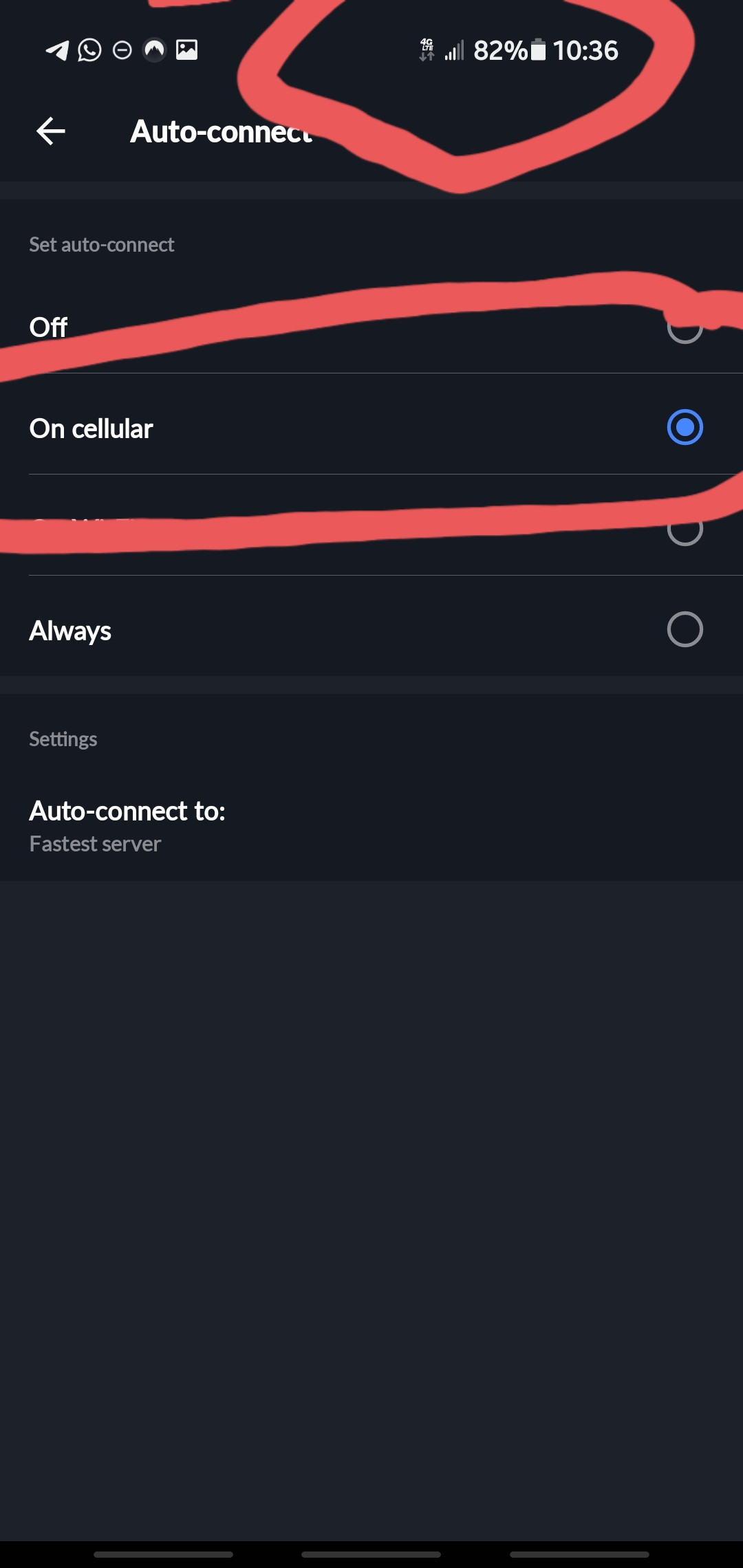This detailed caption describes a screenshot taken from a cell phone displaying network connection settings with annotations made in a red outline:

"The screenshot captures the 'Auto Connect' settings of a cell phone. At the very top, the header displays 'Auto Connect' with a left-pointing arrow next to it. Below this header, in small gray text, it reads 'Set Auto Connect.' Directly beneath, in larger white text, the option 'Off' is displayed, accompanied by an empty gray circle to the far right. Below 'Off,' the option 'On Cellular' is displayed with a filled blue circle to its right. However, there is another word partially obscured by an on-screen annotation.

Further down, the option 'Always' is visible with another empty gray circle similar to the 'Off' circle, followed by the 'Settings' heading. Below 'Settings,' the option 'Auto Connect to Fastest Server' is shown.

Highlights in the screenshot made by a crude finger-drawn annotation in red outline are notable. These annotations encircle the phone icons at the top right of the screen, including the battery percentage, the time, and signal bars, among other details obscured in the screenshot. Additionally, the 'On Cellular' option is outlined in red from the left to the right, emphasizing it.

The red outline annotations and the appearance of the drawn circles suggest the editing was done using a phone's photo editing tool, with the red lines marking important details of the image."